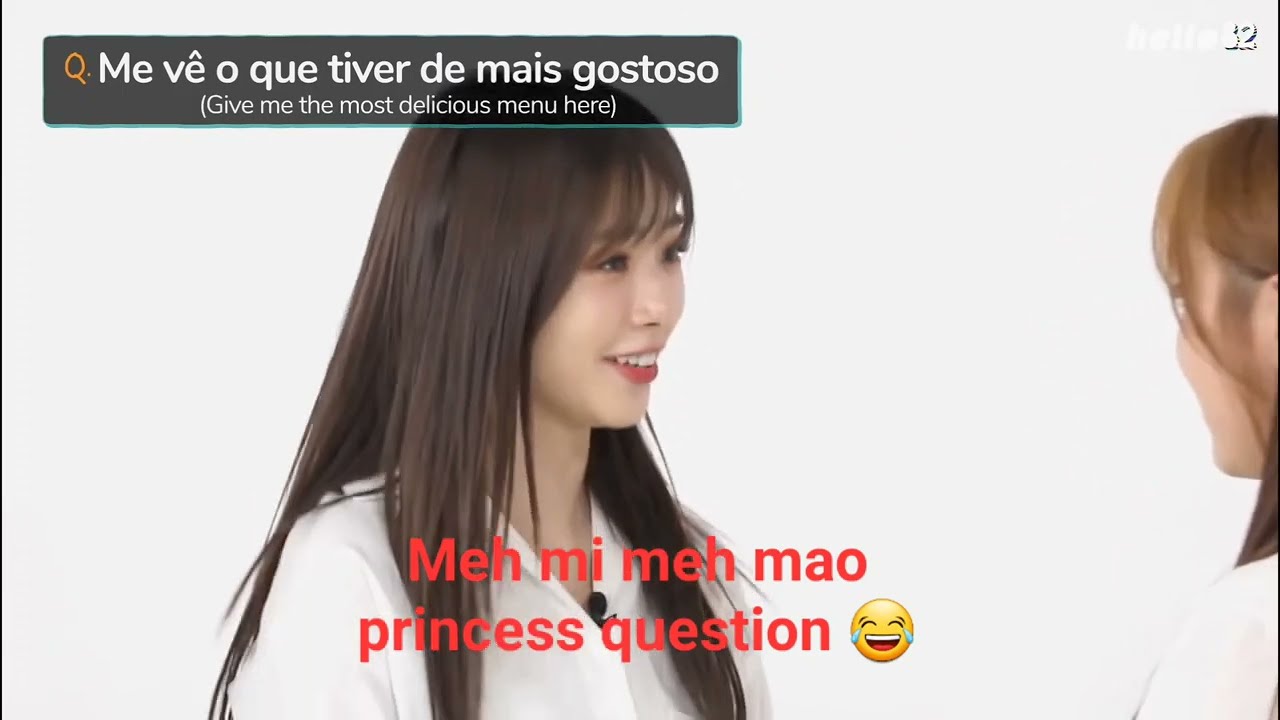The image displays a horizontal rectangular scene featuring two young women of Asian descent engaged in conversation, set against a white background. Both women are smiling warmly. The woman on the left, with long dark brown hair, is wearing a white top and has a microphone clipped to her shirt. The woman on the right has lighter, reddish-brown hair and is also dressed in a white top.

Overlaid text in the middle of the image, in regular red font, reads "M-E-H, M-I MEH MAO," followed by "princess question" and a yellow emoji that is crying and laughing. In the upper left corner, within a transparent gray rectangle with white font, there's a sentence that appears to be in a foreign language: "Me veo que tiber de maiz gostoso, Benissa" which is translated beneath as "give me the most delicious menu here."

The scene exudes a light-hearted and engaging atmosphere, hinting that it might be a still from a TV show or an advertisement.